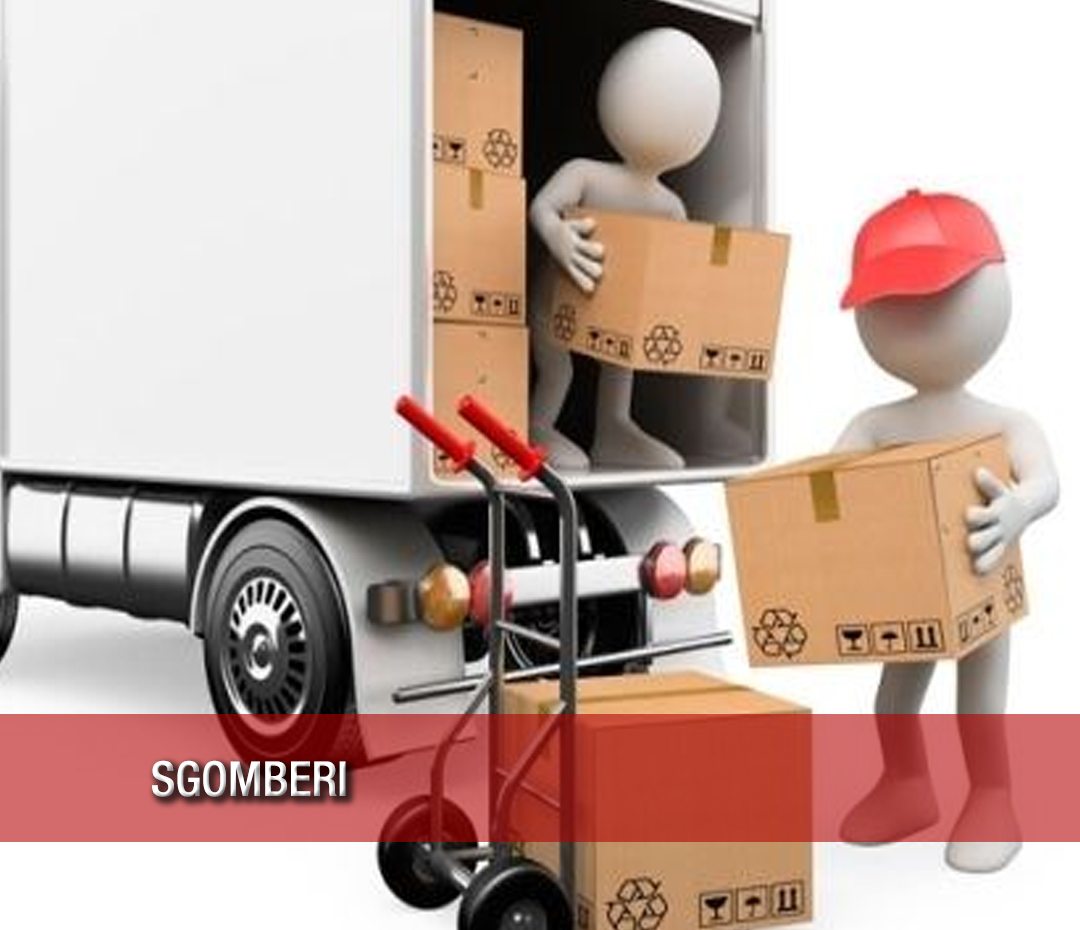The image portrays a digital animation of a moving company scene set against a completely white background. At the top left is a large white box truck with gray and silver accents, inside which a cartoon-style character is positioned, holding a brown package. This character, depicted in white like a toy figure, appears to be maneuvering the package from within the truck's interior, which shows additional brown boxes stacked. On the ground near the truck, another animated character wearing a red hat is handling a brown package, preparing to place it on top of another package that is already positioned on a hand truck with red handles, situated near the bottom of the image. A red banner stretches across the lower section of the image, featuring the white text "S-G-O-M-B-E-R-I." The scene implies an advertisement for a moving company, showcasing colors predominantly of white, gray, silver, brown, red, maroon, and black.